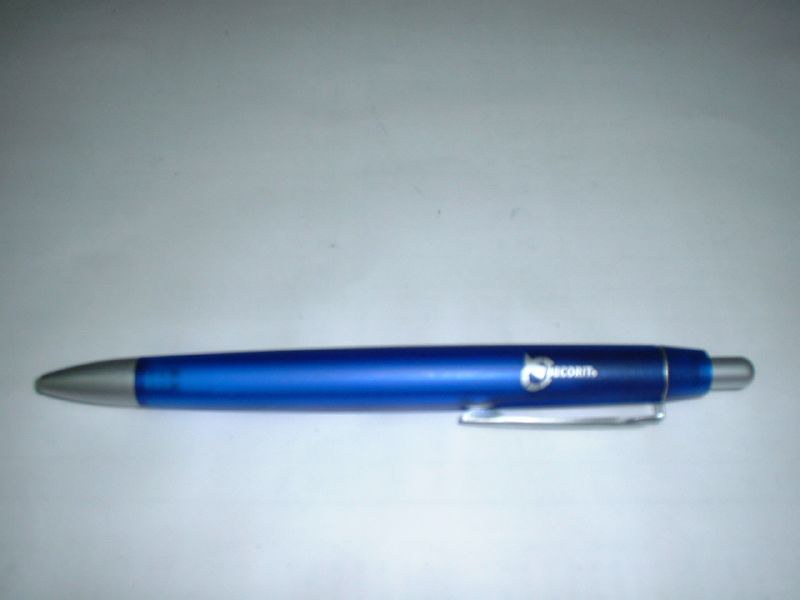The image features a horizontally positioned blue ink pen set against a background that transitions from a light gray at the bottom to a darker gray towards the top. The pen, which is a clicker type, has a thin and somewhat dark blue body. On the left end of the pen is a silver tip cap, and on the right end is a silver button used for extending and retracting the pen's tip. Additionally, the pen includes a silver clip for attaching it to a pocket or notebook. Just to the right of the clip, there is a silver logo and text that appears to be the brand name, reading "Pecoret" with an R trademark symbol beneath it.